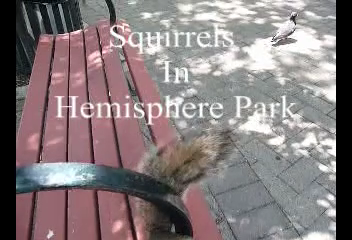In a brightly lit daytime outdoor scene, an image showcases a redwood park bench with wrought iron armrests on each side. The bench, positioned diagonally from the lower right to the upper left portion of the frame, is depicted in profile with its seven vertical wooden slats visible. A gray brick sidewalk in front of the bench sets the background, casting dappled light presumably from an out-of-frame tree. Dominating the center is a partially visible gray and brown squirrel's tail, slightly blurred, emerging from the lower edge and curving behind the iron armrest. The upper right corner features a pigeon facing east. Overlaying the scene in white text are the words: "Squirrels in Hemisphere Park." A slight hint of a black iron trash can is discernible in the lower right corner, adding to the park's atmosphere.